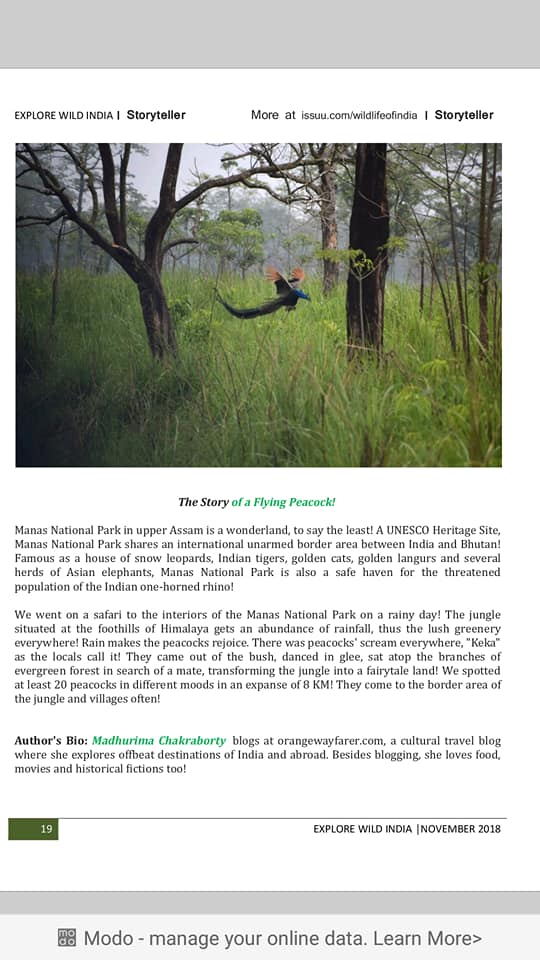Explore Wild India Web Page Overview:

At the very top of the web page for Explore Wild India is a gray square box. Below this, the title "Explore Wild India Storyteller" is displayed prominently, followed by a link to Issues.com stated as "more at Issues.com Wild FEC Find India." 

Further down, a captivating photograph of a dense forest features prominently. You can observe towering trees and long green grass. Within this lush greenery, there's a bird which appears to resemble a peacock. Below the image, the text "The Story" is written in black, and "Of a Flying Peacock" is highlighted in green.

A descriptive paragraph follows, narrating the wonders of Manus National Park, an esteemed UNESCO heritage site possessing a shared international unarmed border with India and Bhutan. The park is celebrated for hosting snow leopards, Indian tigers, golden cats, golden langurs, and large herds of Asian elephants. Importantly, it serves as a sanctuary for Indian one-horned rhinos, a species facing threats. 

The text elaborates on a safari experience in Manus National Park on a rainy day, emphasizing the park's location at the Himalayan foothills, which contributes to its vibrant, lush environment. The narrative vividly portrays the excitement of witnessing peacocks revel in the rain, dancing and calling out as they emerged from the bushes and perched on the branches in search of mates. The scene is described as being almost like a fairy tale, with numerous peacocks (at least 20) observed within an 8-kilometer range.

The author's biography follows, introducing Manda Hurrian Chakraburti, who blogs at orangewayfarer.com, a cultural travel blog dedicated to exploring lesser-known destinations in India and beyond. Besides her passion for blogging, she enjoys food, movies, and historical fiction.

In the left sidebar, the text "Explore Wild India November 2018" appears, followed by two horizontal gray bars. The bottom bar provides a link to "Mondo-Manager Online Data," inviting visitors to learn more.